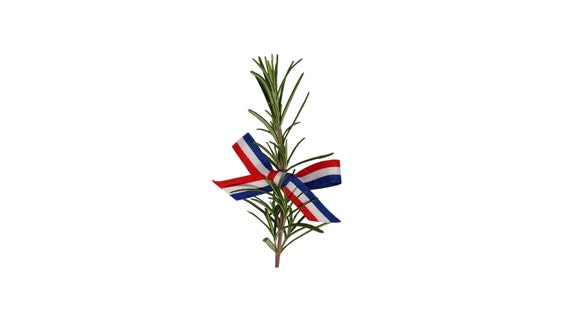The image is a small, vertical photo featuring a single branch that appears to be from a pine tree, identifiable by its thin green needles and a small portion of a brown stem at the bottom. Tied around the middle of this branch is a red, white, and blue ribbon, forming a perfect bow. The ribbon is arranged so that, in one direction, the colors sequence from red at the top to white in the middle and blue at the bottom; in the opposite direction, it transitions from blue to white to red. The bow has a distinct knot in the center, with two loops and trailing ends, all set against a plain white background. The overall composition gives a detailed, almost realistic impression of this festive decoration.